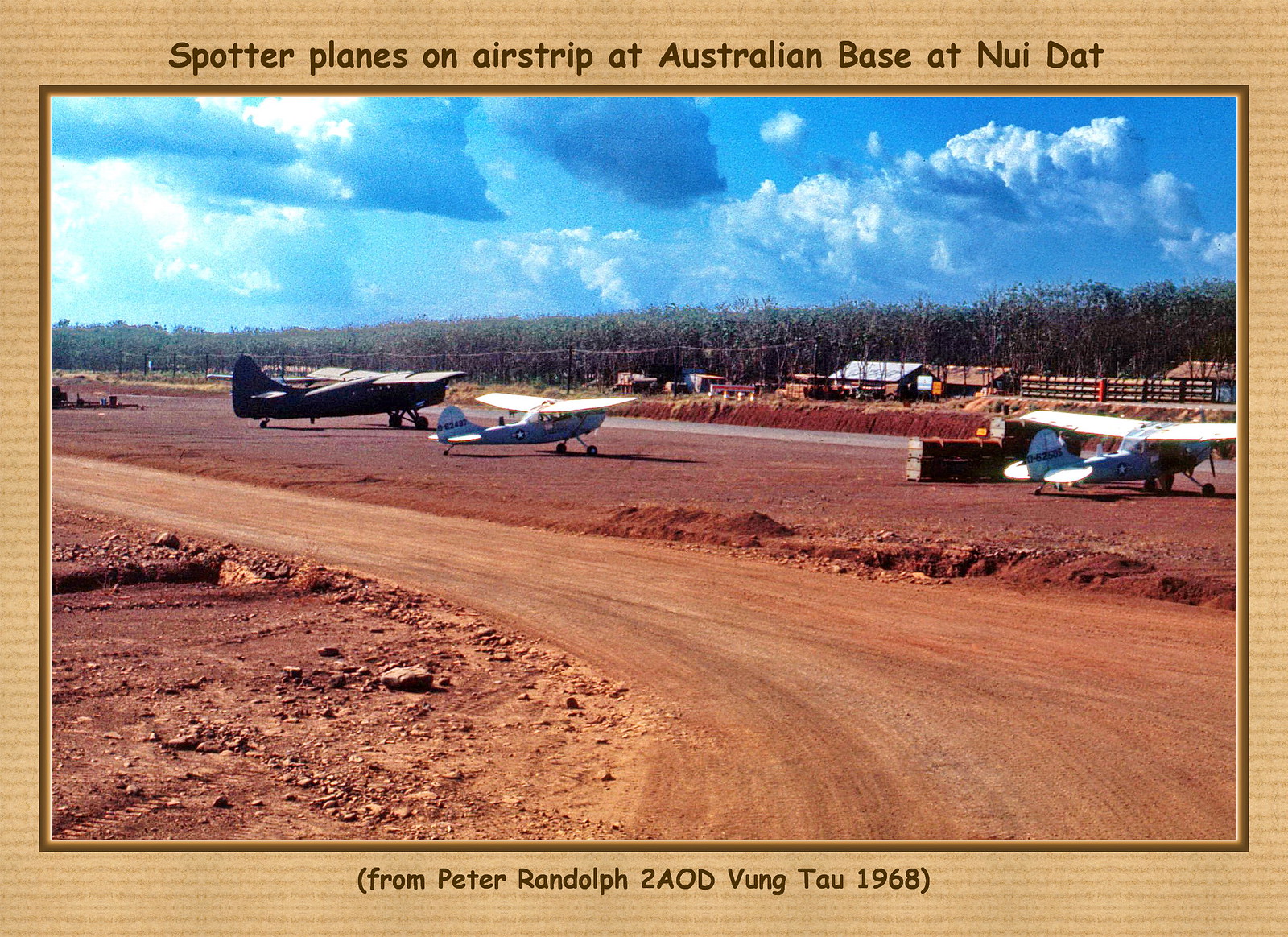This vintage photograph captures an airfield at the Australian base at Nui Dat in 1968, sent from Peter Randolph to AOD Vung Tau. The scene features a central unmetalled path, covered in brown and red soil, stretching across the outdoor area. Situated on the right side of this path are three airplanes—two light blue and one black—all neatly lined up on the ground. The foreground displays the well-traveled dirt road characterized by clay-like surface lumps. In the background, a cluster of log cabins is visible, along with a thick, expansive forest and scattered trees. The sky above is a brilliant blue, filled with clouds, enhancing the serene yet historical ambiance of the airfield. The photograph is framed with a light brown border, bearing the caption, "Spotter planes on airstrip at Australian base at Nui Dat" at the top, and inscribed at the bottom, "From Peter Randolph to AOD, Vung Tau 1968."